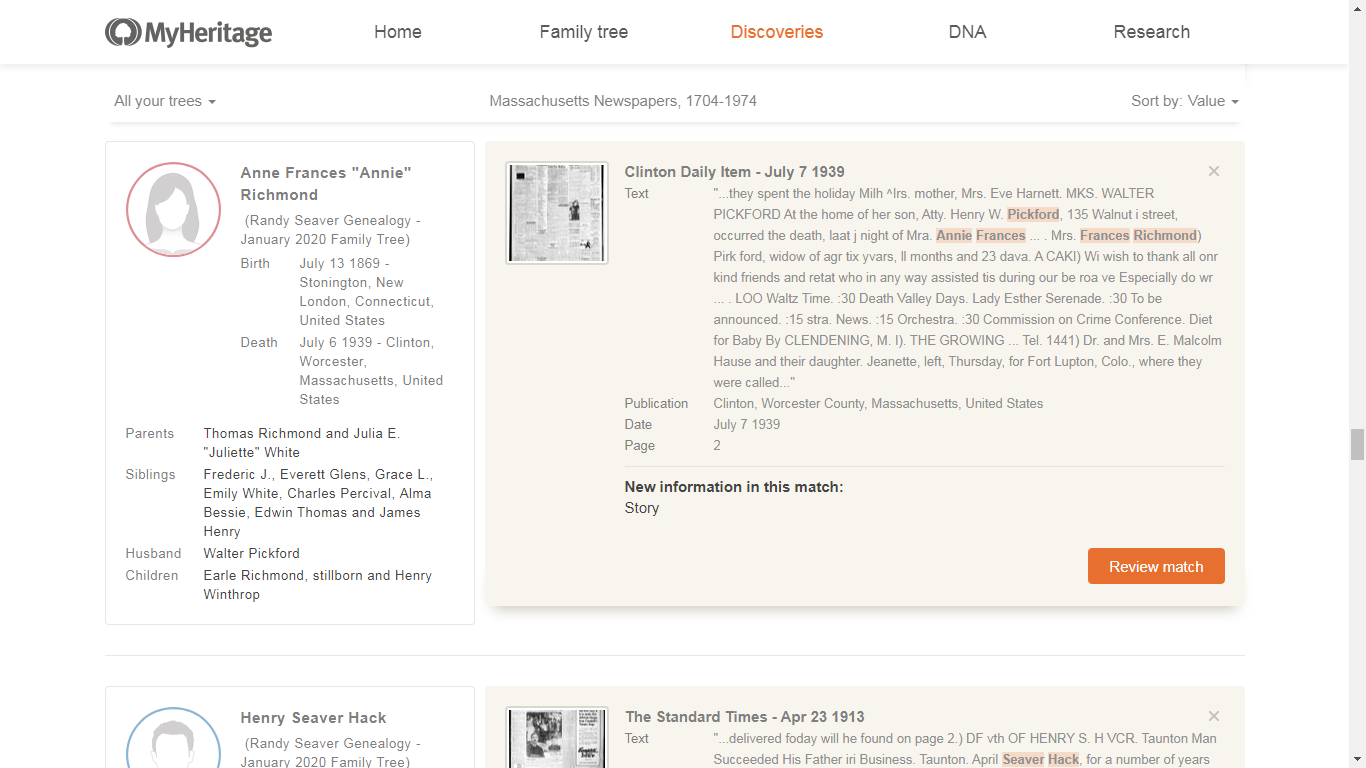This is an image of a webpage from MyHeritage. The website's header features the words "MyHeritage" in black font. The navigation menu includes options such as "Home," "Family Tree," "Discoveries" (highlighted in orange), "DNA," and "Research," all in black writing except for "Discoveries." Below the header, the page displays several text boxes. One box contains a red circle with a grayscale image of a woman. To the right of this, there is a newspaper clipping with numerous words written in gray font. Beneath this section, the text reads "New Information in this Match, Story." An orange rectangular button labeled "Review Match" in white font is also visible.

Another section features a blue circle with a man's picture and the name "Henry Seaver Hack" next to it. There is another newspaper clipping titled "The Standard Times" dated April 23, 1913. A sorting area labeled "Sort by" allows users to select sorting options from a dropdown menu indicated by a down arrow. A scrollbar with up and down arrows is located on the right side of the page.